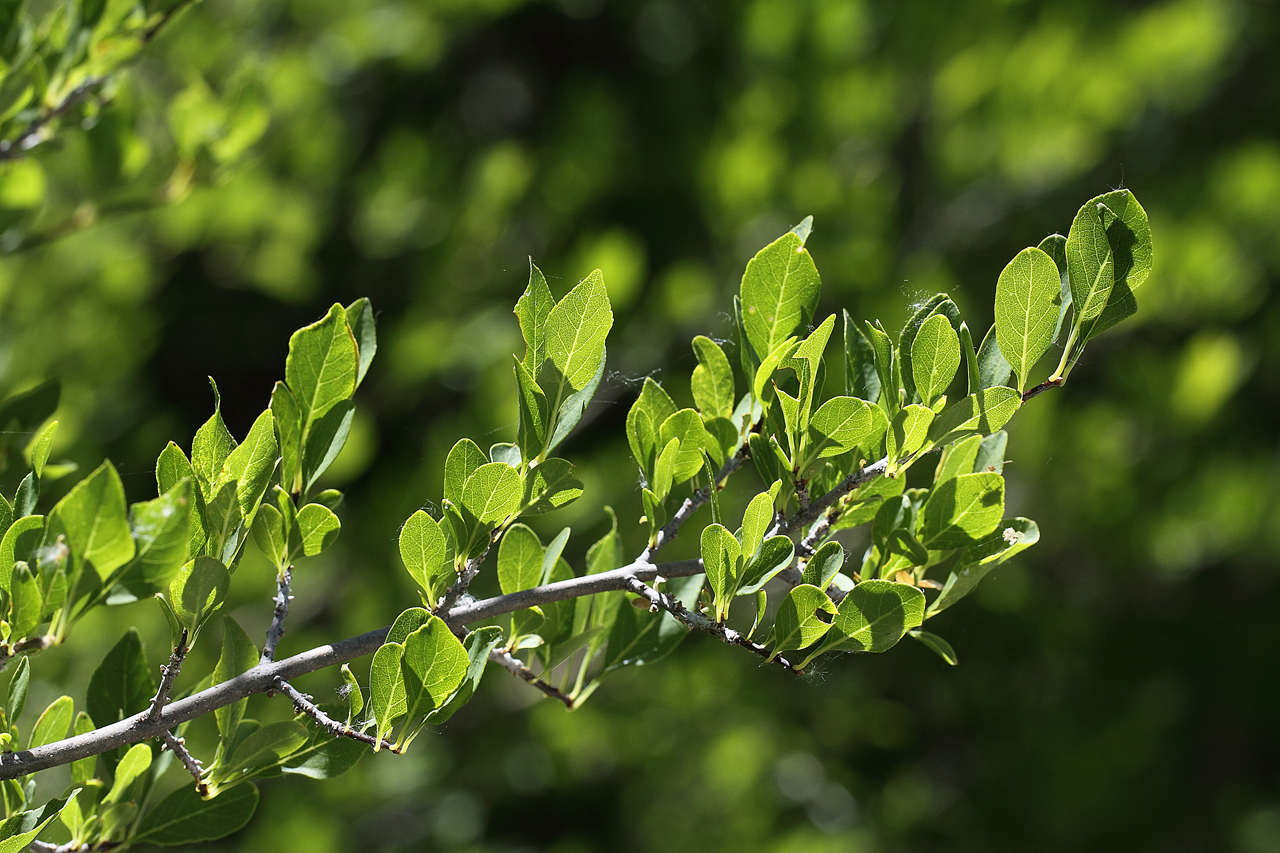A professionally shot, full-color photograph taken outdoors on a sunny day using natural light showcases a nature scene in a horizontally rectangular orientation. The image focuses on a medium-gray colored tree branch extending diagonally from the lower right-hand corner up towards the center right. The branch, featuring numerous smaller twigs adorned with vividly green, oval-shaped leaves, demonstrates the growth pattern typical of a shrub. The leaves, some with slightly triangular tips and others rounded, appear lush and full, catching the sunlight and featuring light green center veins. The entire setting hints at a summer day. The blurred background consists of a blend of greens, blacks, and whites from other out-of-focus plants, emphasizing the sharp, detailed foreground. No people, animals, or text exist in the image, highlighting the serene simplicity of the natural moment captured.